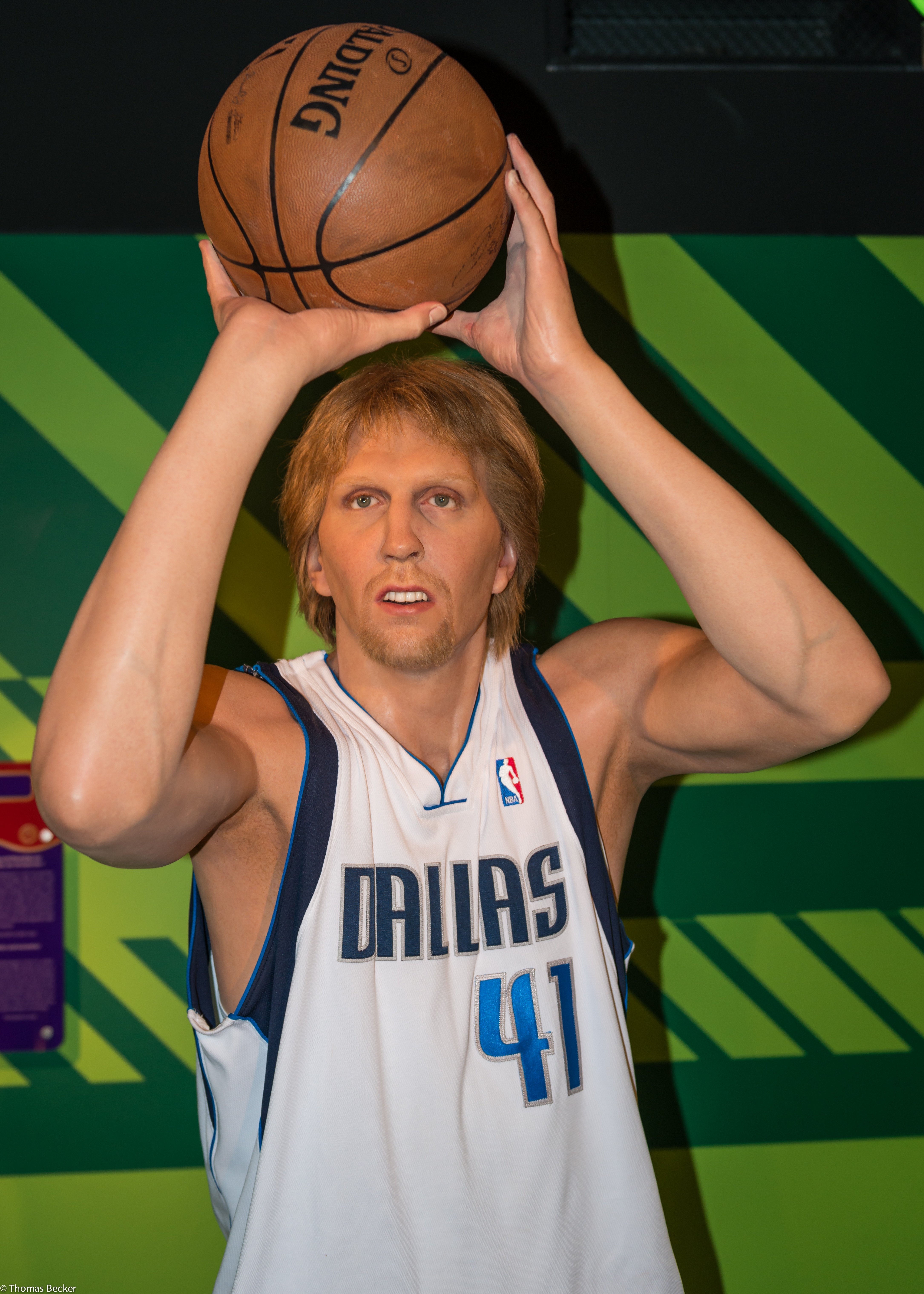This is a highly detailed color photograph featuring a wax sculpture of famed basketball player Dirk Nowitzki from the Dallas Mavericks. The sculpture captures Dirk mid-action, holding a basketball above his head as if preparing to shoot. He is wearing the team’s official jersey, which is white with blue trim. The jersey prominently displays "Dallas" in blue letters and the number "41" in blue as well. He has dirty blonde hair, and his mouth is slightly open, showing his teeth. 

In addition, there is a small NBA logo, colored in red, white, and blue, visible on the upper right of his chest. The background features a striking green design with both light green and dark green stripes, adding depth to the image. A partially readable placard with red, yellow, and purple elements is located towards the lower middle-left of the backdrop. This setting, likely a museum, vividly showcases the sculpture amid an array of colors including lime green, forest green, black, orange, blue, and purple, with the rectangular photograph being vertically oriented.